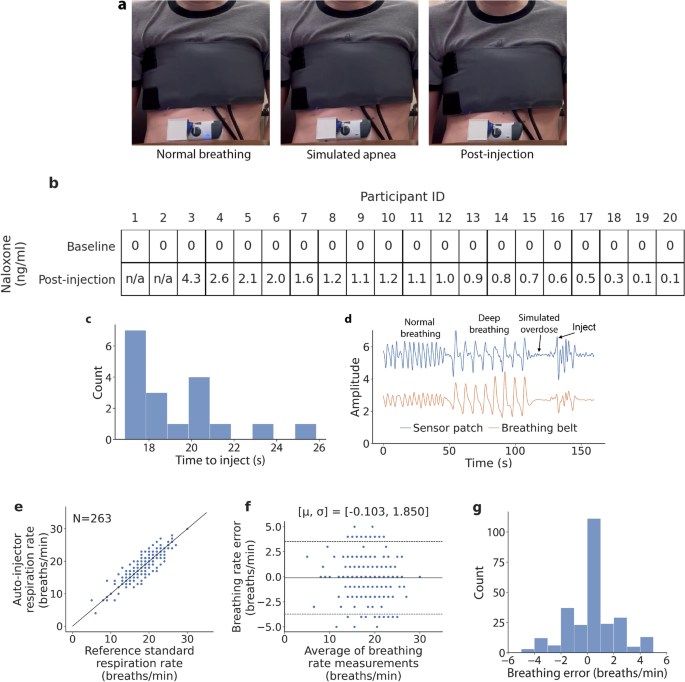The image displays several diagrams and photographs associated with a study on breathing patterns and the effects of an injection. The primary photograph shows a close-up of a Caucasian participant's chest and stomach, with the shirt pulled up to reveal a dark gray underbra. A breathing apparatus is attached to their chest. This main section is divided into three smaller images, each showing different breathing states: "Normal Breathing," "Simulated Apnea," and "Post-Injection."

The image is sectioned into multiple labeled parts:
- **Section A:** Photographs of the participant’s chest labeled with different breathing states: Normal Breathing, Simulated Apnea, and Post-Injection.
- **Section B:** A detailed table listing Participant IDs and their naloxone levels (NG-ML) post-injection. Baseline levels are zero for all participants, while post-injection levels vary.
- **Section C:** A bar graph showing the count versus time to inject, indicating the most common times for injection among participants.
- **Section D:** Monitors displaying breathing patterns with the y-axis labeled as amplitude and the x-axis as time. Diagrams illustrate various breathing states: Normal Breathing, Deep Breathing, Simulated Overdose, and the state Post-Injection.
- **Section E:** A line graph plotting the reference standard respiration rate against the auto-injector respiration rate, showing a direct correlation.
- **Section F:** Another plot graph detailing the breathing rate error compared to the average breathing rate measurements.
- **Section G:** A bar graph showing the relationship between breathing rate error and count, indicating that higher counts correlate with lower breathing errors.

Overall, the image provides a comprehensive visual representation of a study on breathing patterns, detailing various states of breathing under different conditions, as well as the quantitative data from multiple participants before and after injection.